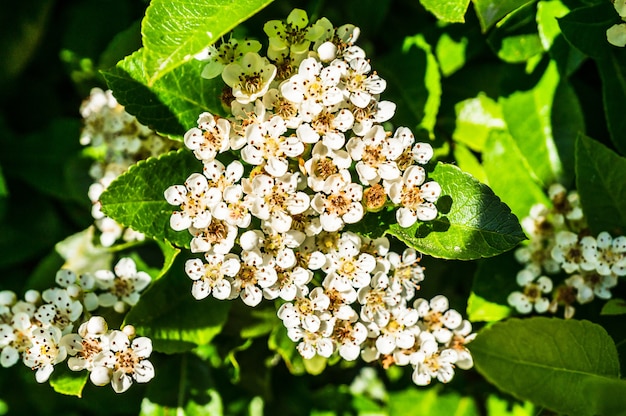This high-resolution photograph showcases an up-close view of a flowering plant with an impressive cluster of tiny white flowers, each flower prominently featuring five delicate petals dotted with faint specks. The petals frame a central yellow or golden core, lending a honeysuckle-like appearance. The image's focal point is a central grouping of around 25 such flowers, with other clusters visible in the shaded background, indicating a dense, healthy bloom.

The leaves of the plant are lush green and teardrop or oval-shaped, broad relative to the small flowers. They range from darker shades in the shadows to lighter areas where sunlight directly hits, highlighting the plant's vibrant health and absence of disease or insect damage.

Additional details, like the mix of light and shadow playing across the scene, vary across the image, with the central cluster fully illuminated, showcasing their pristine condition. Overall, this well-focused photograph captures the serene beauty and intricate details of the flowering plant, presumably growing in a pot or planter.